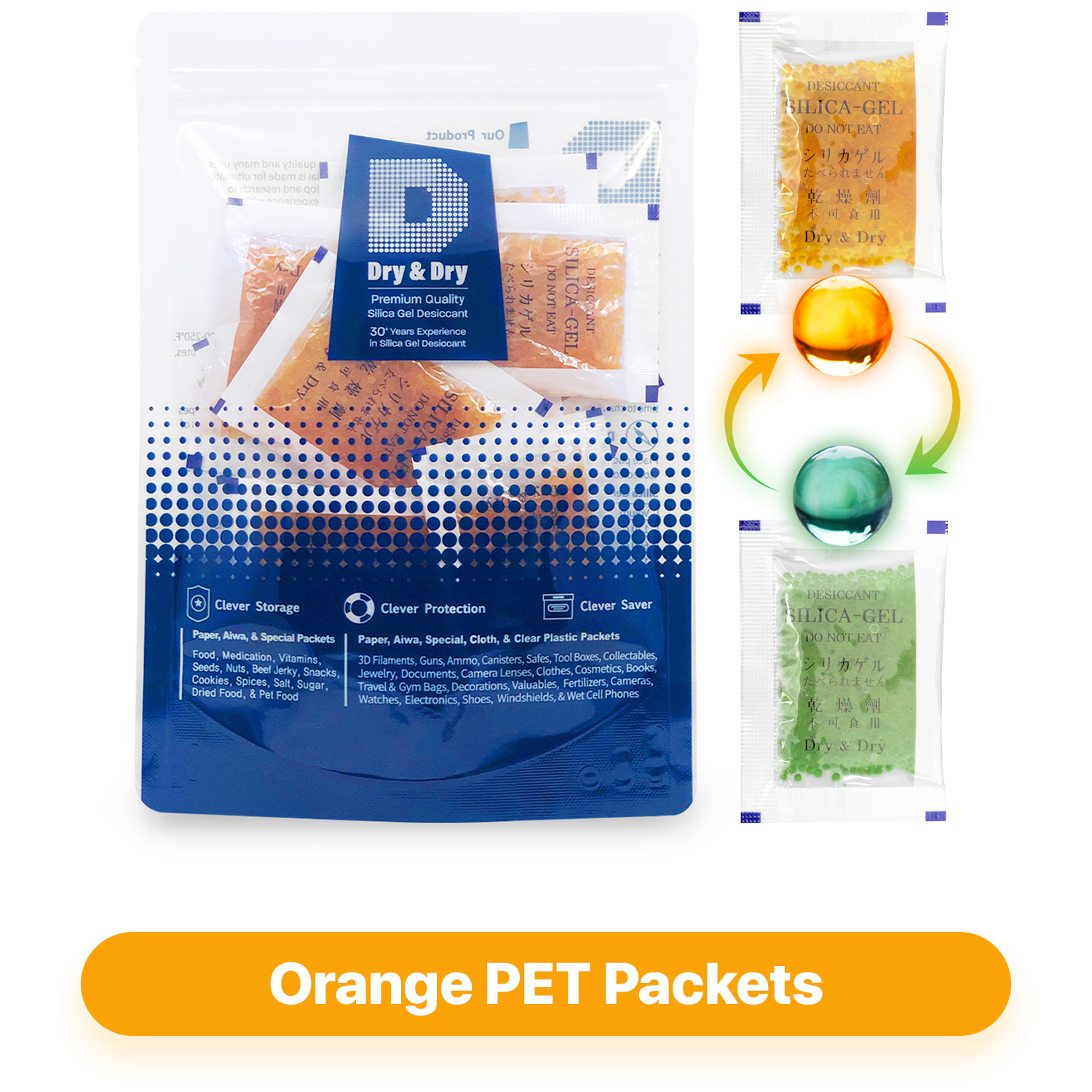The image displays a collection of silica gel packets organized with detailed labeling and color coding. At the bottom, an oblong orange packet with rounded ends bears the title "Orange Pet Packets." Above this, positioned to the left side of the image, there is a large clear Ziploc bag labeled "Dry & Dry," featuring slogans like "clever storage," "clever protection," and "clever saver." The bag contains numerous smaller packets of silica gel, ranging in colors and types. Each small packet is labeled "Silica Gel," promoting its premium quality with "30 years experience." To the right of this large bag, there are two individual silica gel packets: the one on top contains brown silica gel, while the one below it contains green silica gel. Between these two individual packets, there are small colored balls, with a yellow ball located between the upper and lower packets and a green ball situated below that. The text within the image mentions the versatile applications of silica gel in preserving items like food, medicine, and pet products. The colors featured prominently include orange, green, blue, and clear hues, emphasizing the varied and specialized nature of the silica gel packets.